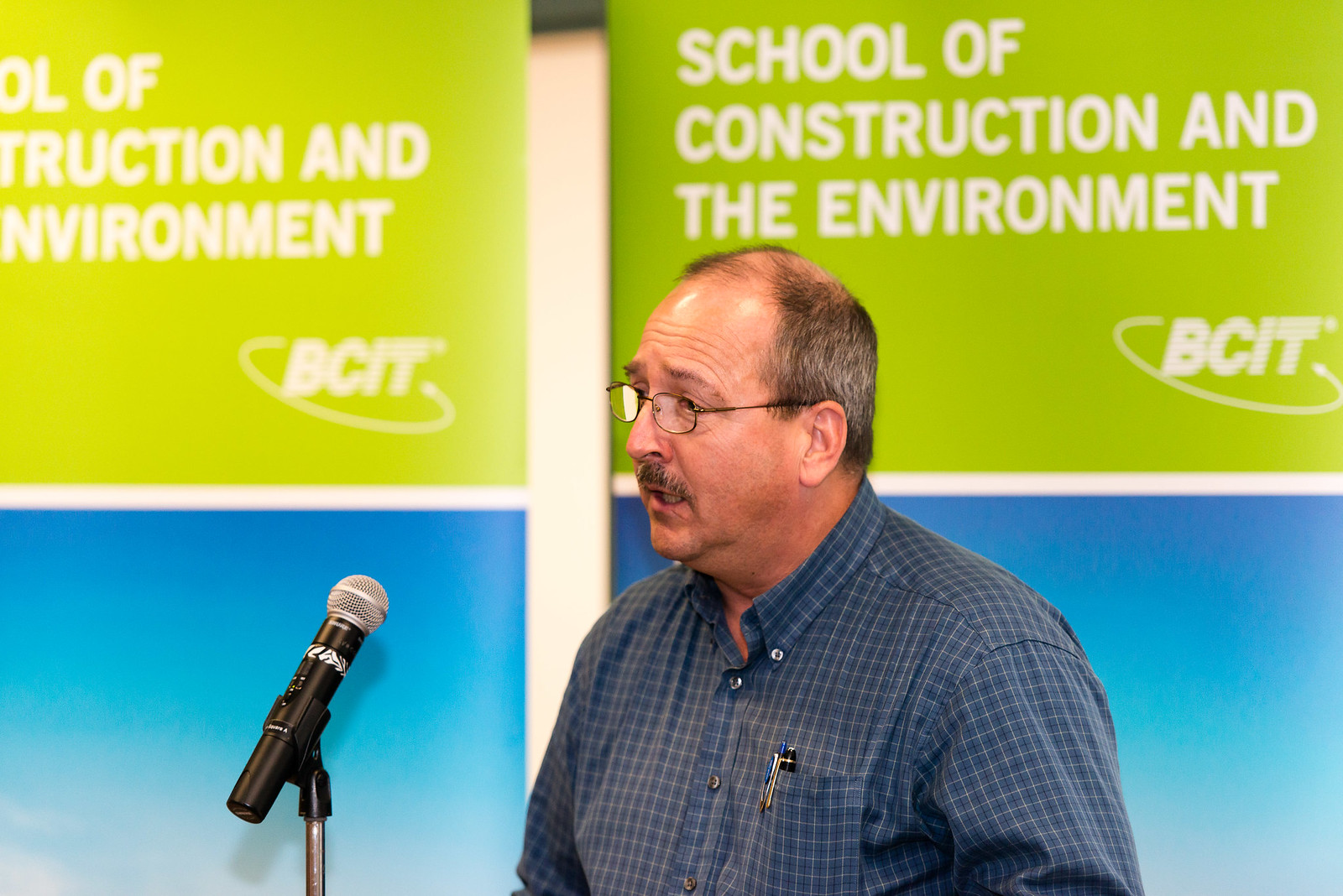The image depicts a close-up of a white man speaking into a large black microphone with a silver round piece mounted on a stand to the left side of the frame. He is wearing a blue and white checked button-down collared shirt with a couple of pens in the front pocket. He has a small or thin brown mustache, and his hair is partially bald on top, with a mix of gray and brown on the sides and back. He is wearing small wired glasses and facing towards the left, with his mouth open as if in mid-speech. 

The blurred background features a wall sectioned into two colors: blue on the bottom and green on top, separated by a horizontal white stripe. The top green section contains white text that reads "SCHOOL OF CONSTRUCTION AND THE ENVIRONMENT" in all caps, left-aligned. In the lower right-hand corner of the green section, there is a logo with the text "BCIT" accompanied by an angled swirl around it. This setting suggests that the man is giving a presentation or speech related to the School of Construction and the Environment.